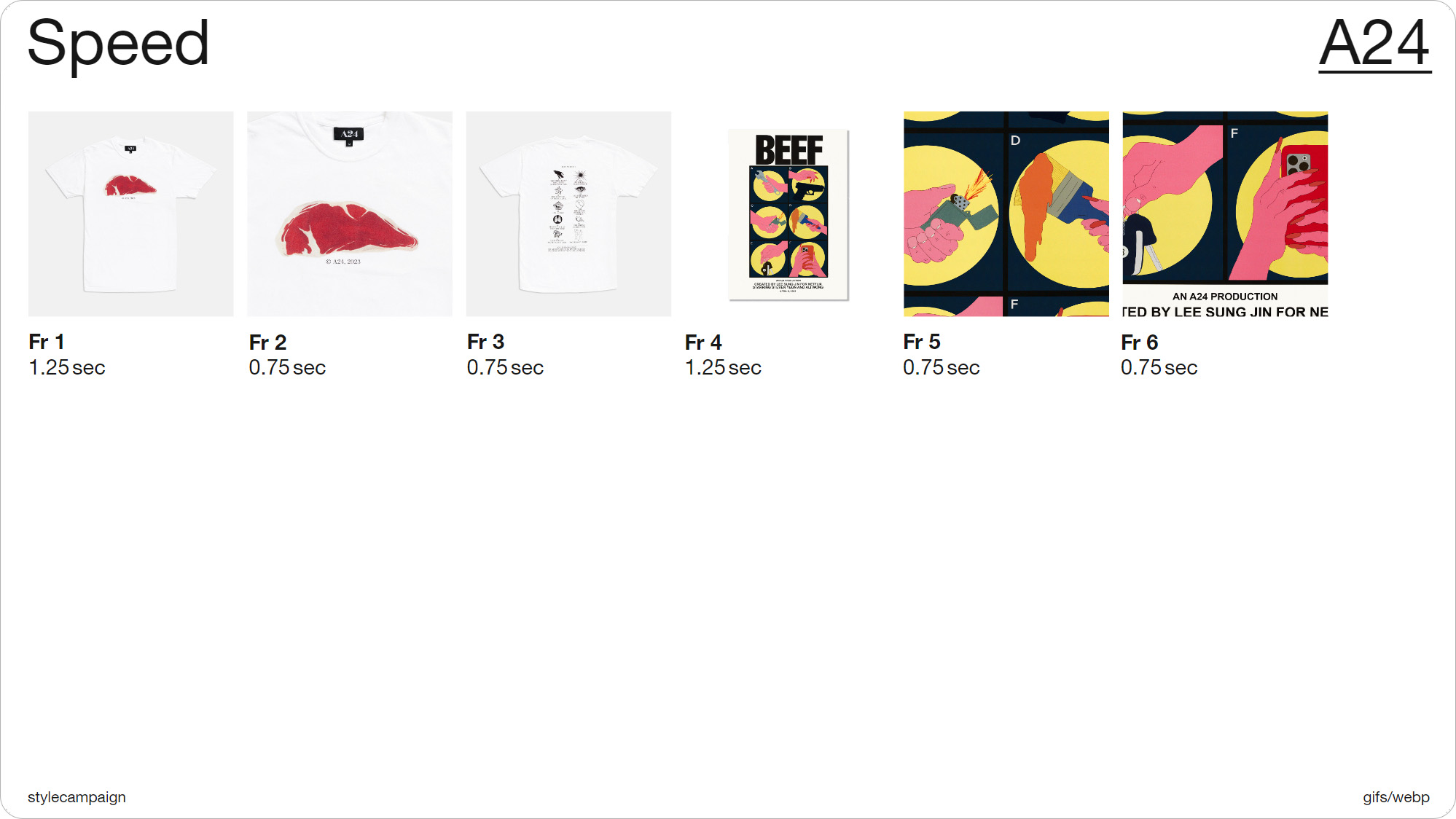This screenshot displays a screen with six evenly sized thumbnails, likely representing different products. At the top, the word "Speed" is positioned to the left, while "A24," underlined, is located on the right. Below this header, six thumbnails are arranged in a row, labeled FR1 through FR6 from left to right. Underneath the row of thumbnails, there is a mention of "time in seconds."

- **FR1**: Features a white t-shirt adorned with a red design.
- **FR2**: Provides a close-up view of the red design on the white t-shirt from FR1.
- **FR3**: Displays another white t-shirt, this time with a different graphic design.
- **FR4**: Shows a poster with the word "Beef" prominently displayed. The poster has a black background and features yellow circles.

Each element is distinct and structured in a way that highlights the visual details and categorization of the thumbnails.